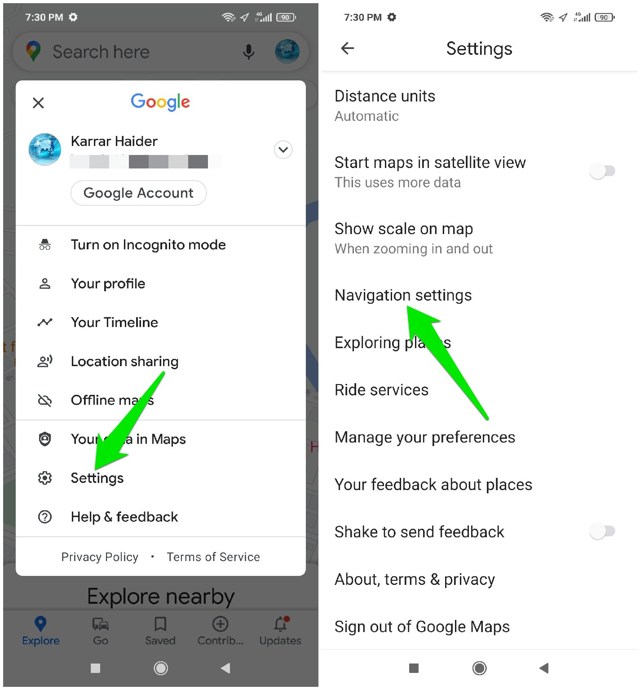The image displays two screenshots of a Google settings page on a cell phone. The left screenshot forms the background, showing the outline of the cell phone with a light black background. In the foreground, a white horizontal rectangular box prominently features the Google logo at the top center.

Below the logo, the account name "Karar Hater" is displayed, indicating it is the user's personal account. Directly under the name is the "Google Account" button, followed by several options:

1. Turn on Incognito Mode
2. Your Profile
3. Your Timeline
4. Location Sharing
5. Offline Maps
6. Your Places
7. Settings (highlighted by a large green arrow)

At the bottom of this box, the options "Help and Feedback," "Privacy Policy" (bottom left), and "Terms of Service" (bottom right) are visible.

The second screenshot is overlaid on the right side. At the top middle, it reads "Settings." The following options are listed below:

1. Distance Units (in black) with "Automatic" (in light gray) underneath.
2. Start Maps in Satellite View (in black) with an explanatory note "This uses more data" (in gray) and an off-toggle button to the right.
3. Show Scale on Map (in black) with "When zooming in and out" (in gray) underneath.
4. Navigation Settings (in black), highlighted by a large green arrow.
5. Exploring (partially covered by the green arrow).
6. Ride Services
7. Manage Preferences
8. Your Feedback About Places
9. Shake to Send Feedback
10. About Terms and Privacy

At the bottom, the options include "Sign Out of Google Maps." The page bottom shows a black square on the left, a circle in the middle, and a left-facing arrow on the bottom right.